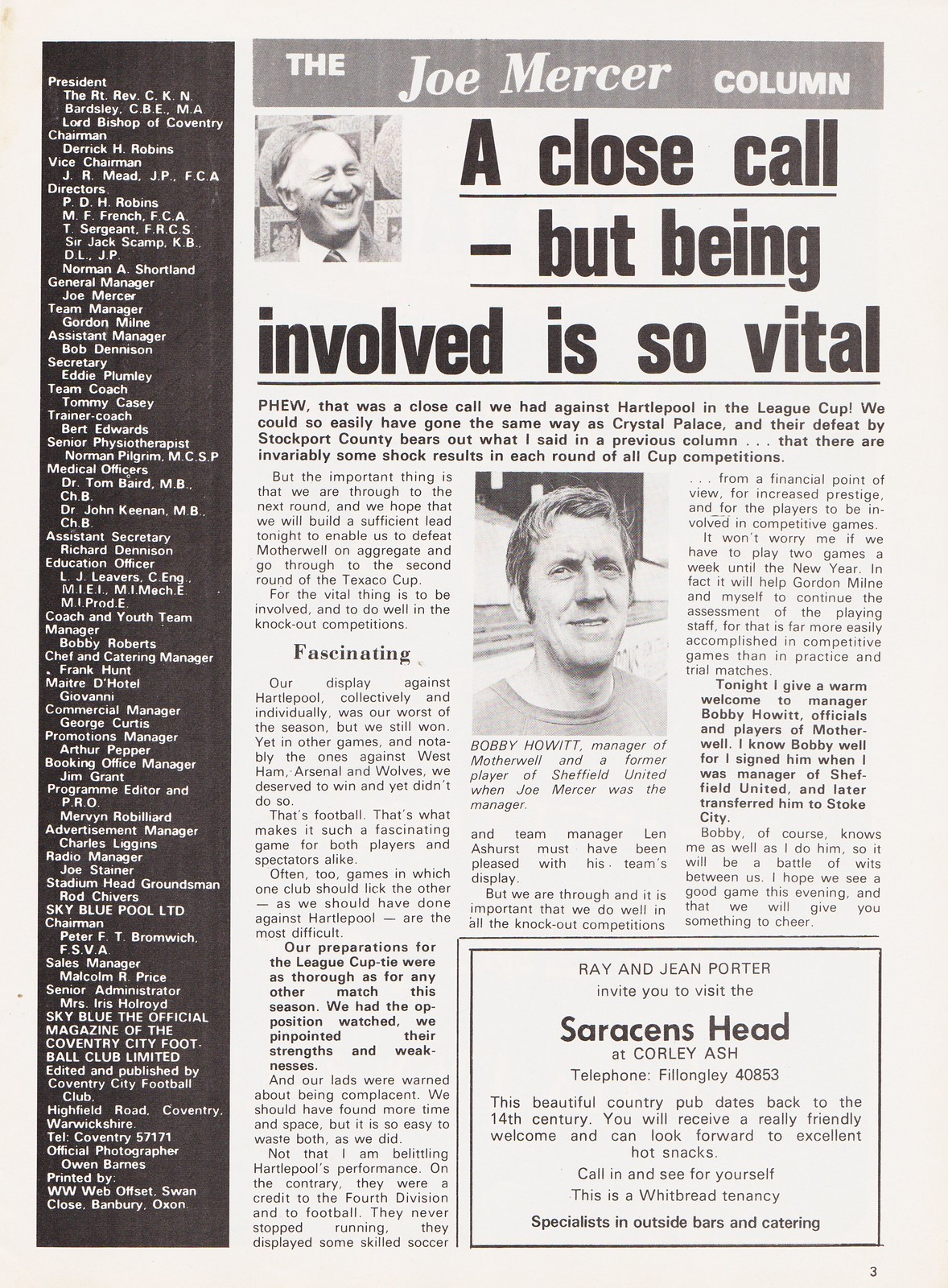This appears to be a scan of a faded, vintage magazine page, likely from a soccer fanzine dedicated to an English soccer club. The page has two main sections: a left vertical black band with white text listing the club's corporate positions, such as president, chairman, vice chairman, directors, and general manager, and a prominent right section featuring "The Joe Mercer Column." At the top of the right section, there's a gray banner reading "MUH" in bold caps, followed by "Joe Mercer" in regular font and "COLUMN" in caps. The main headline of the column, written in big black letters, is "A Close Call - But Being Involved Is So Vital." To the left of the headline is a photograph of Joe Mercer, likely a man in his late 50s or early 60s, with a receding hairline and a big grin on his face. Below the headline, there are three columns of text, discussing topics such as the League Cup, although the print is too small to read clearly. In the middle of the column, there's another headshot of a player, possibly named Rodney Nesbitt, though the caption is difficult to decipher. The lower right-hand corner of the page features an advertisement for "Saracens Head" located at Copley Ash, likely an inn or restaurant, with the names Ray and Jean Porter mentioned along with an invitation to visit.